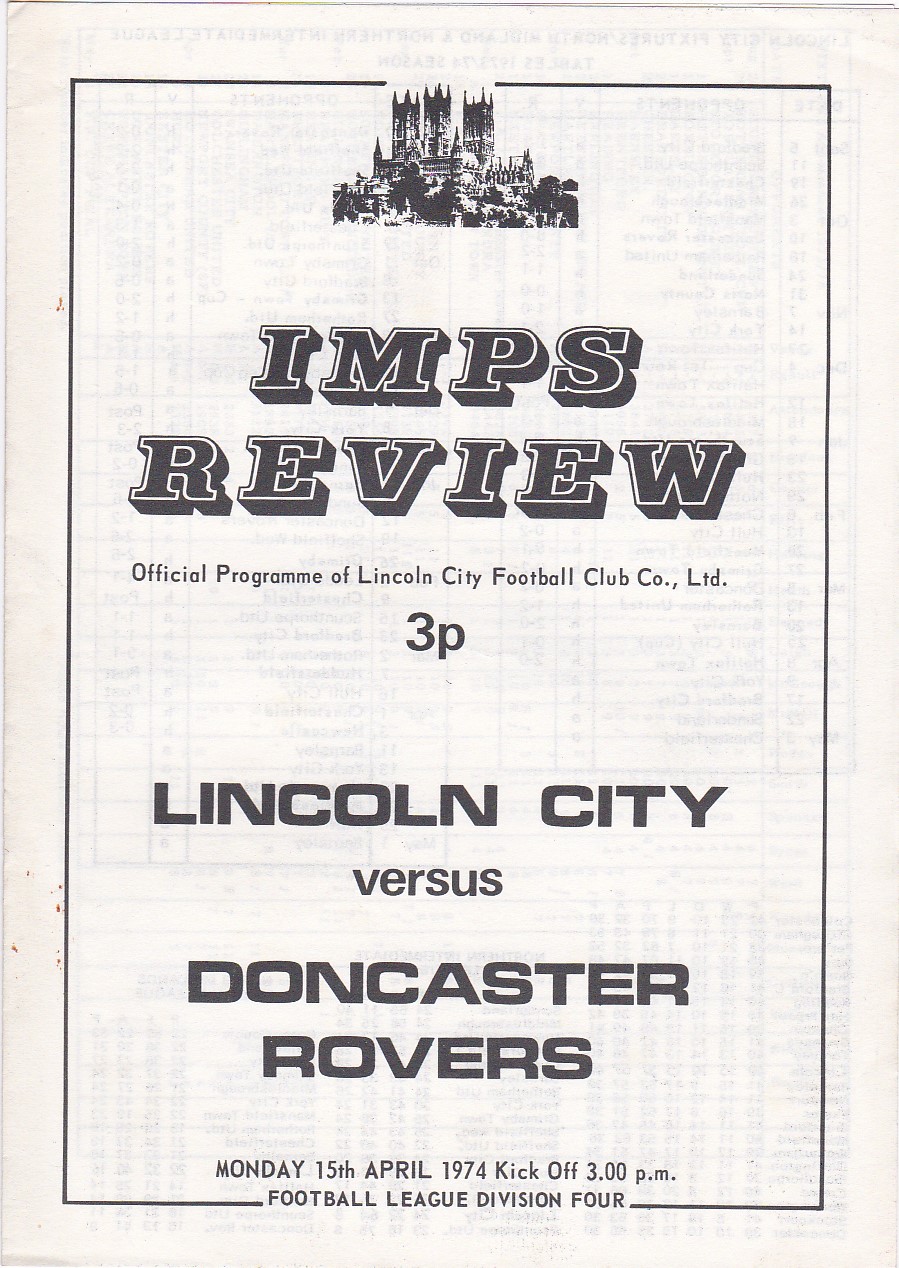The image depicts a game program set against a beige background with a thin black outline. At the top, there's a highly detailed but small sketch of a castle. Below this, bold, capitalized black text outlined in white with a 3D black shadow reads "IMPS REVIEW". Beneath it, in very small print, the text states, "Official Program of Lincoln City Football Club Co. LTD.” Following this, "3P" is displayed, indicating the price. In heavy black capitals, "LINCOLN CITY" is prominently featured. Below this, in smaller black print, the word "Versus" is followed by "DONCASTER ROVERS" in large, black, bold letters. At the bottom, the finer details are given: "Monday, 15th April, 1974, kickoff 3 pm." It concludes with "Football League Division IV."